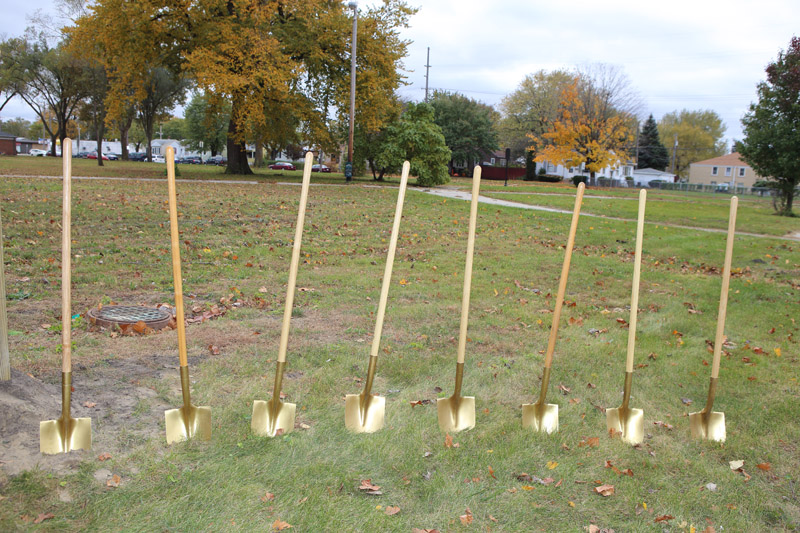This vibrant outdoor photograph, taken in bright daylight, captures a row of eight golden ceremonial shovels with wooden handles, partially pressed into a field of short grass. The shovels, standing upright with their gleaming spades embedded in the ground, dominate the lower half of the image. Positioned for what appears to be a groundbreaking ceremony, they create a striking contrast against the green blades of grass. 

In the background, to the left, a fully grown tree with leaves turning yellowish-green signals the onset of autumn, while to the right, homes and trees already bare of leaves indicate the seasonal transition. A manhole cover is visible on the left side, and a cement path runs through the middle of the image. Further back, a few buildings and possibly some trailer homes, along with scattered vehicles, add layers to the setting. The scene is an elegantly composed snapshot of a moment set to commemorate new beginnings.